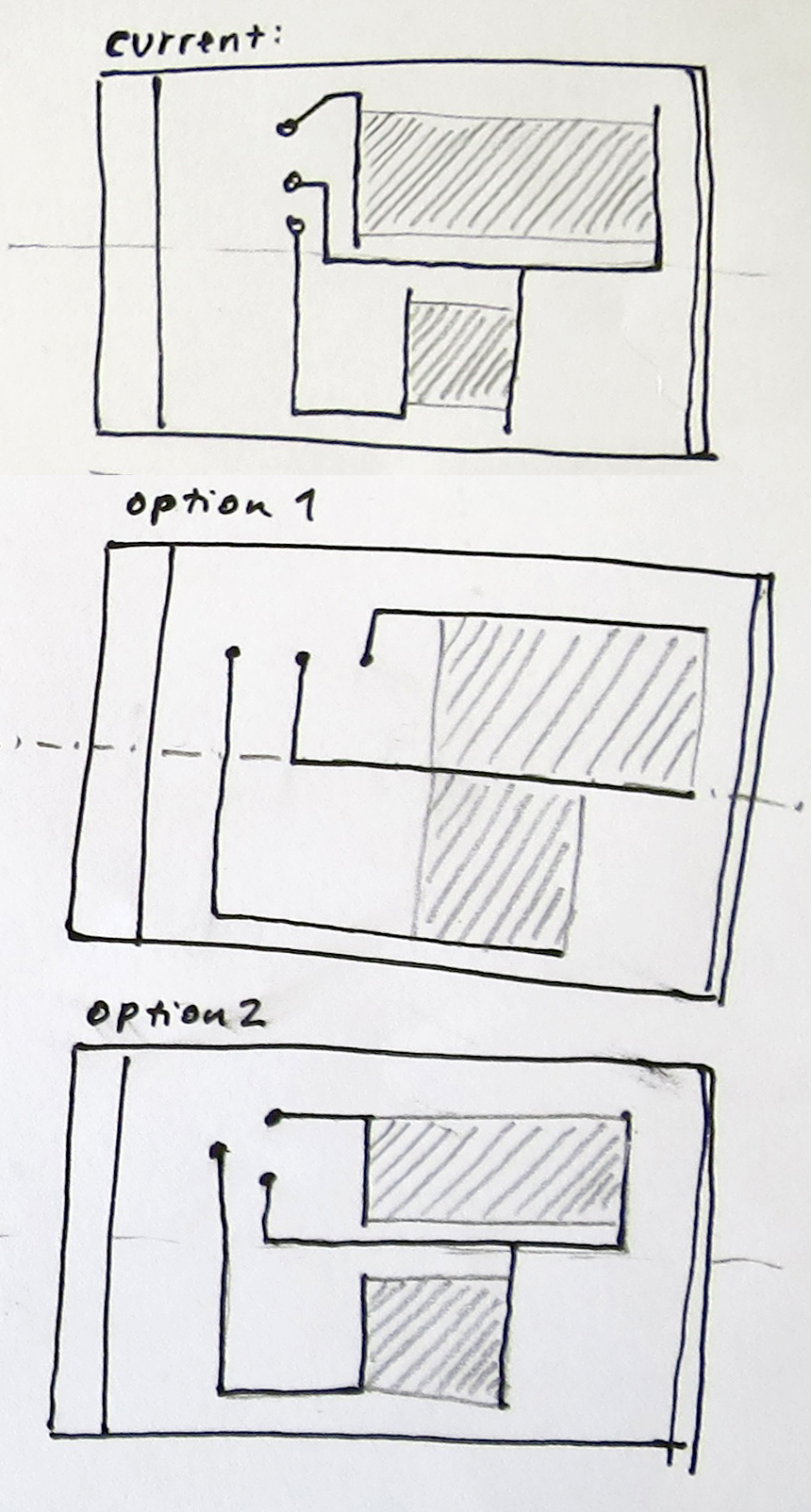This image depicts a piece of paper featuring three detailed illustrations, each presenting different configurations for constructing barriers or structures within a defined space. All drawings are meticulously rendered in black pen and ink.

The common elements across all three illustrations include a large rectangular boundary containing smaller geometric shapes—a rectangle and a square. These shapes are strategically positioned differently in each option to explore various spatial arrangements.

- **Current Configuration:** The rectangle is centrally located within the larger rectangle, with a small gap below it. The square is centered directly underneath this gap.
- **Option 1:** The rectangle is shifted towards the right-hand side of the larger rectangle's boundary. The square is aligned flush with the left edge of the rectangle, creating a close connection between the two shapes.
- **Option 2:** Similar to the current configuration, the square is separated from the rectangle, maintaining an independent placement.

Additionally, several thin lines illustrate potential pathways connecting these shapes, suggesting different movement or flow possibilities within the space depending on each configuration. The intricate detail in the drawings captures the thoughtful consideration given to the spatial arrangement and potential functional relationships between the shapes.